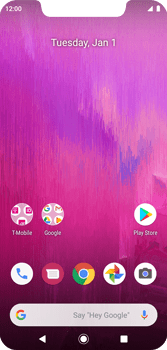This image is a screenshot of a cell phone display, giving the impression of a plastic cover due to its clarity and details. The display frame is notably absent, revealing an indented section at the top center, which is the space where the speaker or earpiece is usually located. 

In the upper left-hand corner of the screen, the time is displayed as 12:00. On the opposite upper right-hand side, the battery icon and the cell phone reception icon can be seen. The wallpaper features a gradient of colors transitioning from black at the bottom to red, then blue, and finally to a pinkish-purplish hue towards the top.

At the bottom of the screen, several app icons are arranged in a row. From left to right, the visible icons are T-Mobile, Google, Play Store, Phone, Messenger, Google Chrome, Photos, and Camera.